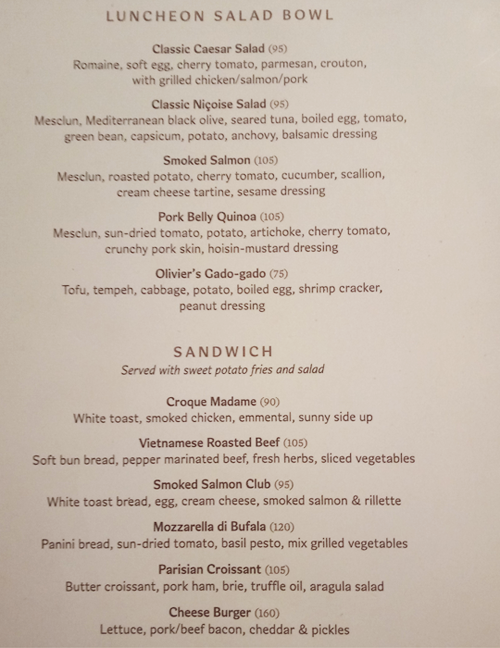The menu is presented in portrait mode, featuring a light tan background with slightly darker brown lettering. The items and names are centered, with dish names in bold and descriptions in a lighter font. At the top, the heading reads "Luncheon Salad Bowl." There are five different salad bowls: Classic Caesar Salad (95), Classic Niçoise Salad (95), Smoked Salmon (105), Pork Belly Quinoa (105), and Oliver's Gado Gado (75). Below the salad section is a list of six sandwiches, all served with sweet potato fries and salad: Croque Madame (90), Vietnamese Roasted Beef (105), Smoked Salmon Club (95), Mozzarella di Bufala (120), Persian Croissant (105), and Cheeseburger (160). The numbers next to each dish likely represent prices, although the currency is not specified and may indicate it's from a non-American locale.